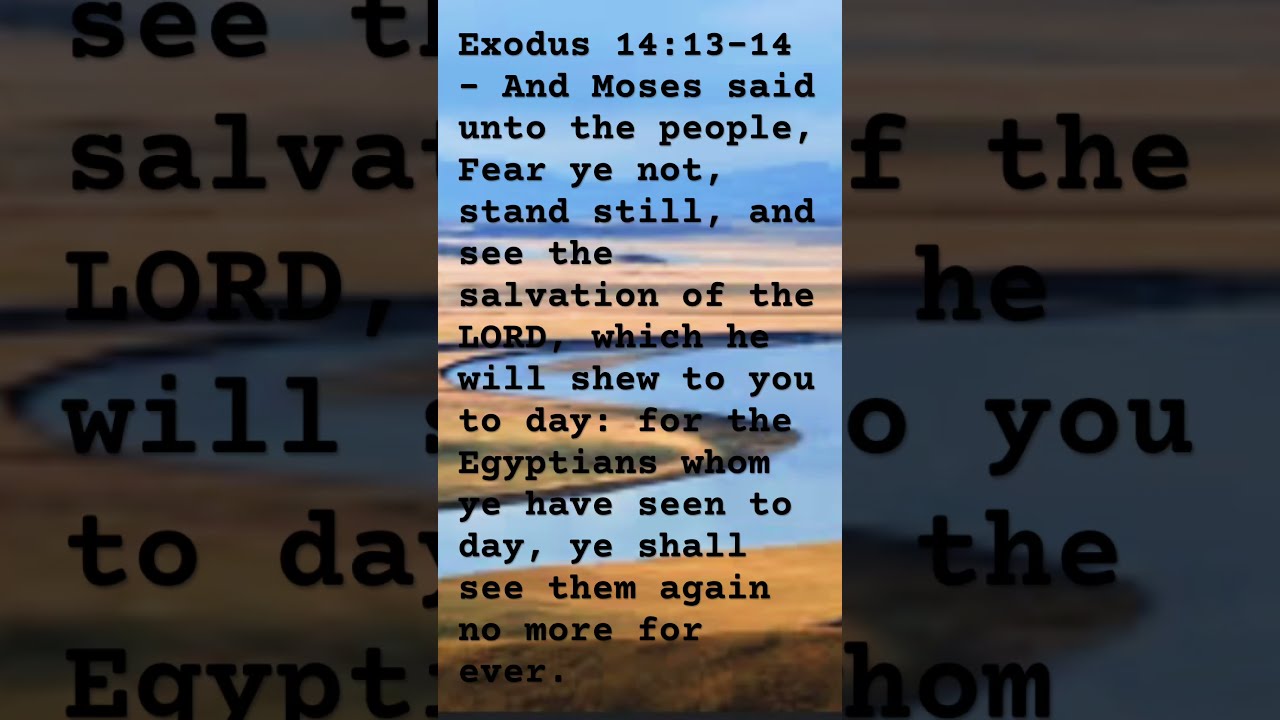The image consists of a computer-generated, vertical landscape featuring a large river snaking across the foreground, surrounded by rolling brown and golden terrain, with the silhouettes of a distant mountain range set against a hazy blue sky. Superimposed over this background is a Bible passage from Exodus 14:13-14, rendered in black text. The central panel of the image clearly displays the scripture, reading, "And Moses said unto the people, Fear ye not, stand still, and see the salvation of the Lord, which he will shew you today. For the Egyptians whom ye have seen today, ye shall see them again no more forever." Additionally, this central panel is flanked by two side panels that magnify portions of the text, highlighting fragments like "salvation," "Lord," "today," and "Egypt." The overall effect blurs and integrates the textual and visual elements, creating a piece of art rather than a conventional photograph.